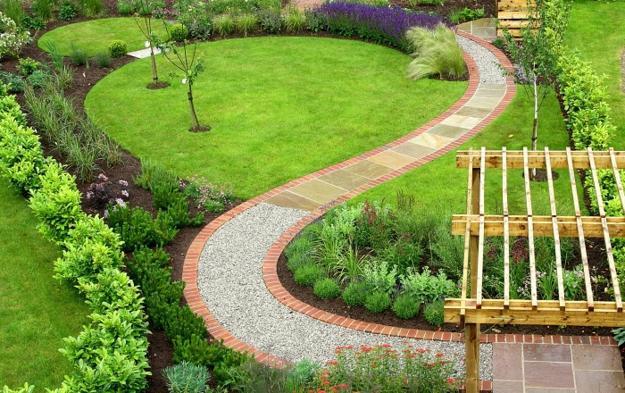This high-angle, daytime aerial shot, likely taken from a drone, captures an exquisitely maintained garden or courtyard area. Dominating the bottom right corner is a wooden trellis or awning that shelters a patio-like space. Extending from this area is a winding gravel and brick pathway, curving through the property like a delicate stream. The pathway, bordered by pink bricks, features a mix of small stones and rectangular marbles in the middle. As it meanders to the right, it passes meticulously cared-for patches of vibrant green grass arranged in circular patterns. These grassy areas are surrounded by lush flower beds filled with a variety of young plants, though none have yet blossomed. Bright and verdant, the entire landscape is punctuated with a few newly planted trees and dense clusters of plants and shrubs. In the distance, a hedge adorned with purple flowers adds a burst of color, enhancing the picturesque beauty of this carefully curated outdoor space.